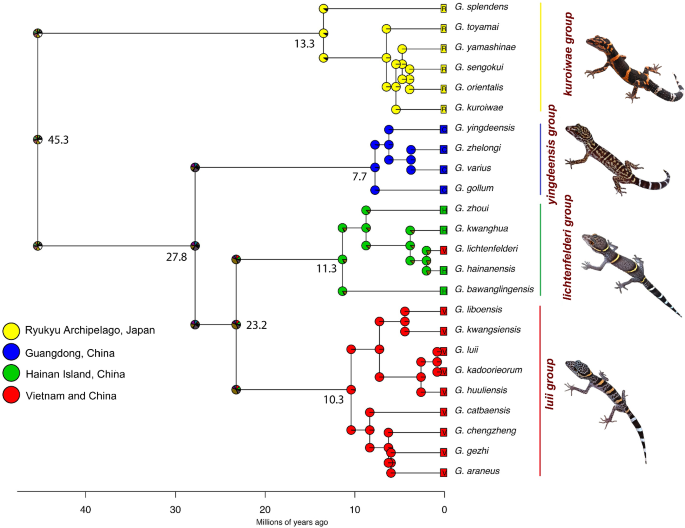This detailed diagram illustrates the evolutionary branching of various reptile species, likely salamanders, over millions of years. Set against a white background, the diagram features a time scale along the bottom, ranging from 0 to 45.3 million years ago from right to left. 

In the bottom left corner, a color-coded legend indicates different geographical regions: yellow for Ryukyu Archipelago, Japan, blue for Guangdong, China, green for Hainan Island, China, and red for Vietnam and China. These colors are used to differentiate the species' origins and their evolutionary paths.

The diagram shows several branching points at significant intervals—45.3, 27.8, and 23.2 million years ago—leading to around 20 distinct species or subspecies. Each branch is color-coded according to its geographical origin. To the right, four main groups are displayed, each corresponding to the color legend: Kuriwai group (yellow), Yangtze group (blue), Lichtenfelderi group (green), and Luli group (red). Accompanying these groups are images of the salamanders, each sharing a similar body shape but with unique markings.

The diagram provides a comprehensive view of how these species diversified and adapted in their respective regions, showcasing both their evolutionary timelines and geographical distributions.